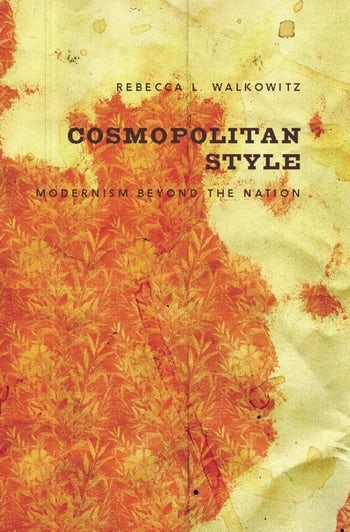The book cover titled "Cosmopolitan Style" by Rebecca L. Walkowitz features an intriguing design. The background primarily consists of a mix of orange and yellow hues, resembling an array of autumn leaves and tree branches, which give the impression of plants tinged with an orange hue instead of their natural green. The background also has a light, almost white section interspersed with what looks like coffee stains or intentional marks, adding a textured and aged appearance, somewhat like a crumpled piece of paper. The title "Cosmopolitan Style" is bold and written in all caps, using a typewriter font where "Style" is aligned right-justified with "Cosmopolitan," so the letters 'E' in "Style" and 'N' in "Cosmopolitan" align precisely. Beneath the bold title, in a smaller, lighter font, the subtitle reads "Modernism Beyond the Nation." The arrangement of colors and text, along with the detailed, textured background, creates a visually engaging and distinctive book cover.